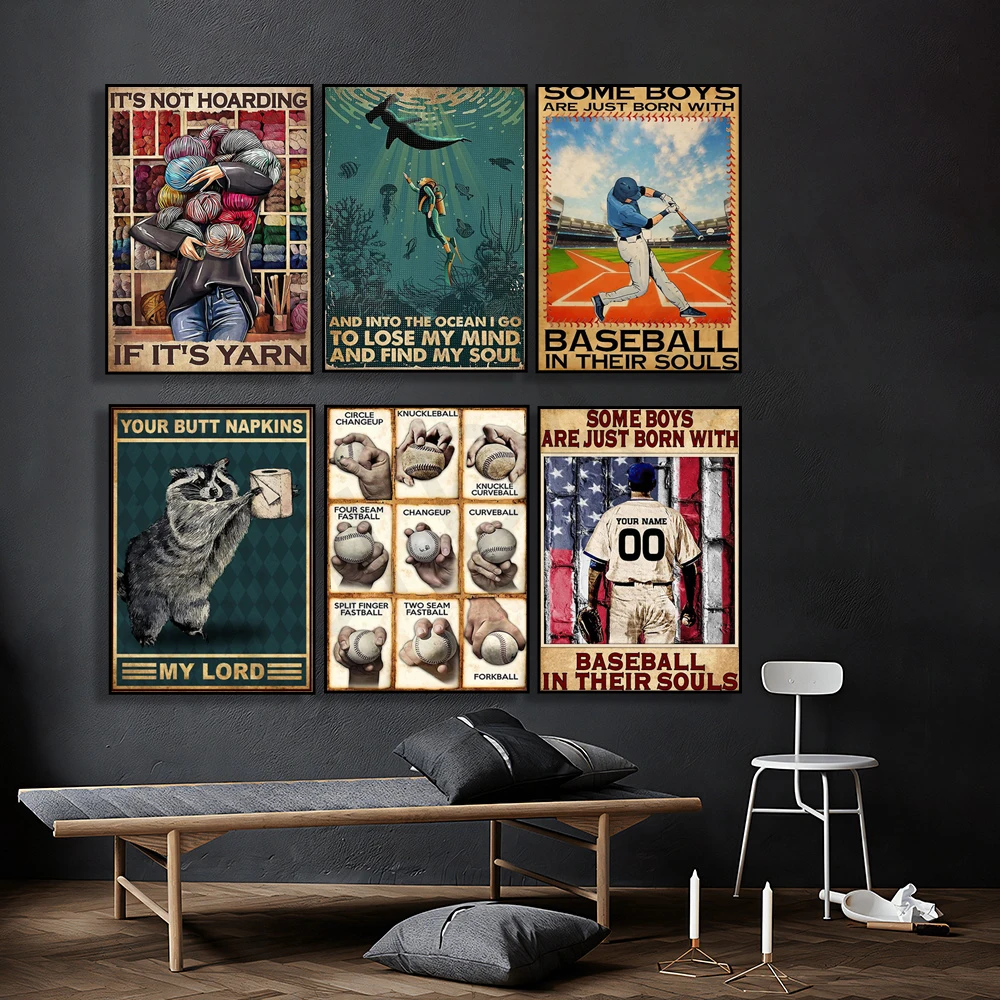The room features a hardwood floor with a gray-accented camp-style bed situated on the floor, adorned with a couple of gray pillows. To the left of the bed, a compact white metal chair with a small backrest stands out. Two slender white candles are positioned on the floor in front of the bed, accompanied by a gray pillow and a white dustpan with a little broom beside them.

The back wall of the room is painted gray and showcases an array of six vividly colored framed posters arranged in two rows of three. From left to right on the top row: a yarn-themed poster with the text "It's not hoarding if it's yarn," an image of a girl diving with a shark overhead captioned "And into the ocean I go to lose my mind and find my soul," and a baseball-themed poster depicting a boy swinging a bat with the words "Some boys are just born with baseball in their souls."

On the bottom row, from left to right: a whimsical raccoon clutching toilet paper with the humorous phrase "You're butt knackings my lord," another baseball poster whose text is unidentifiable, and a patriotic image of a man in a baseball uniform facing an American flag, again with the phrase "Some boys are just born with baseball in their souls." The overall ambiance is modern, with eclectic art that adds personality to the space.